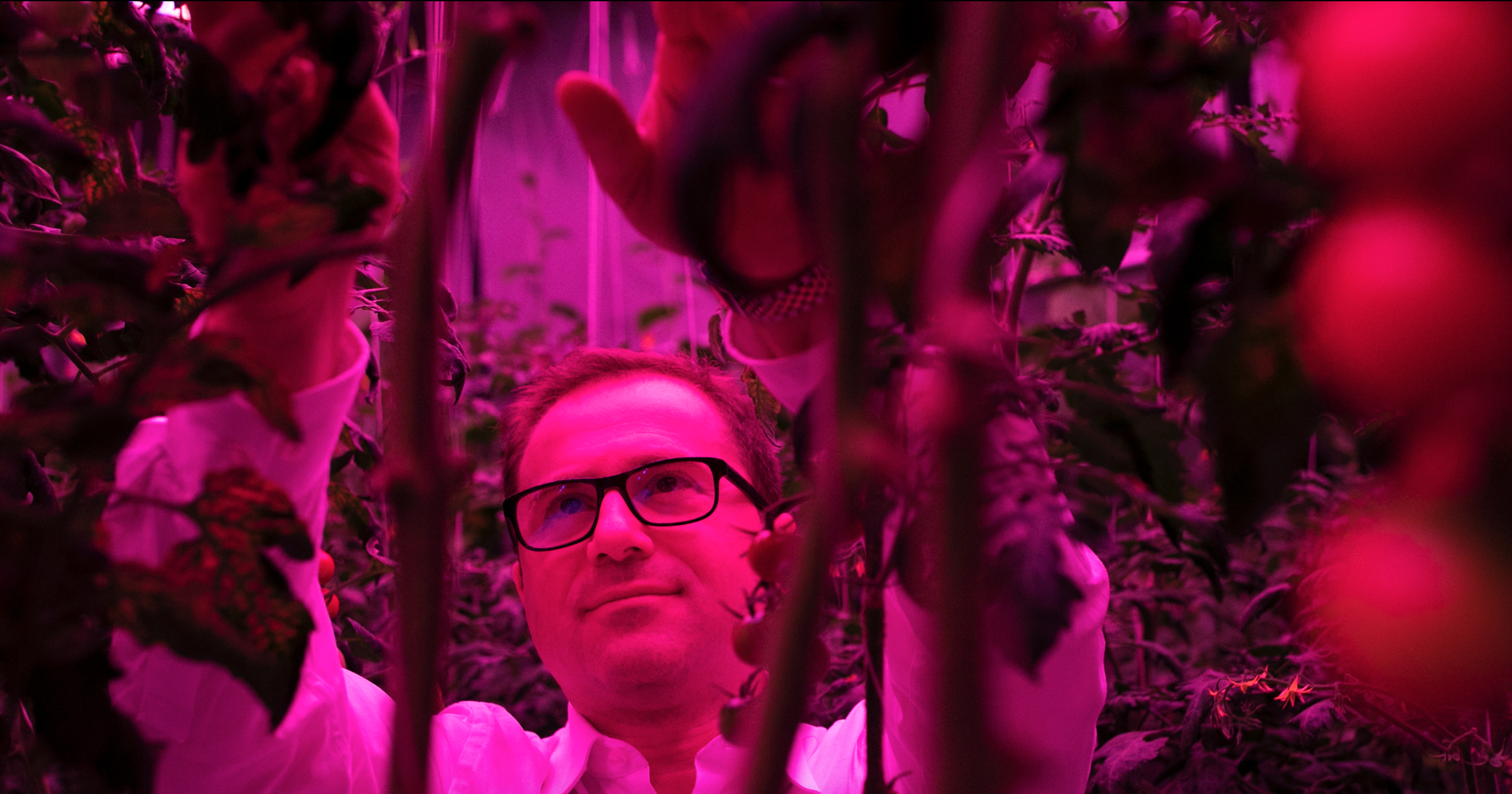In the photograph, a man, possibly a scientist, stands amidst a lush environment, likely a greenhouse, with a distinct red tint enveloping the entire scene. Donning black glasses and a white long-sleeve shirt, his short hair complements his thoughtful demeanor as he appears to engage with the surrounding flora. The foreground captures blurred images of three circular fruits, possibly tomatoes, colored a vibrant orange or red, along with leaves and branches that partially obscure the view. The background faintly reveals elements typical of a greenhouse, such as plastic foil that might be used for isolating environments and capturing heat, enhancing the atmosphere's red and pink hues. This detailed shot focuses on the man, while the surrounding foliage and fruits create a vivid and immersive botanical setting.